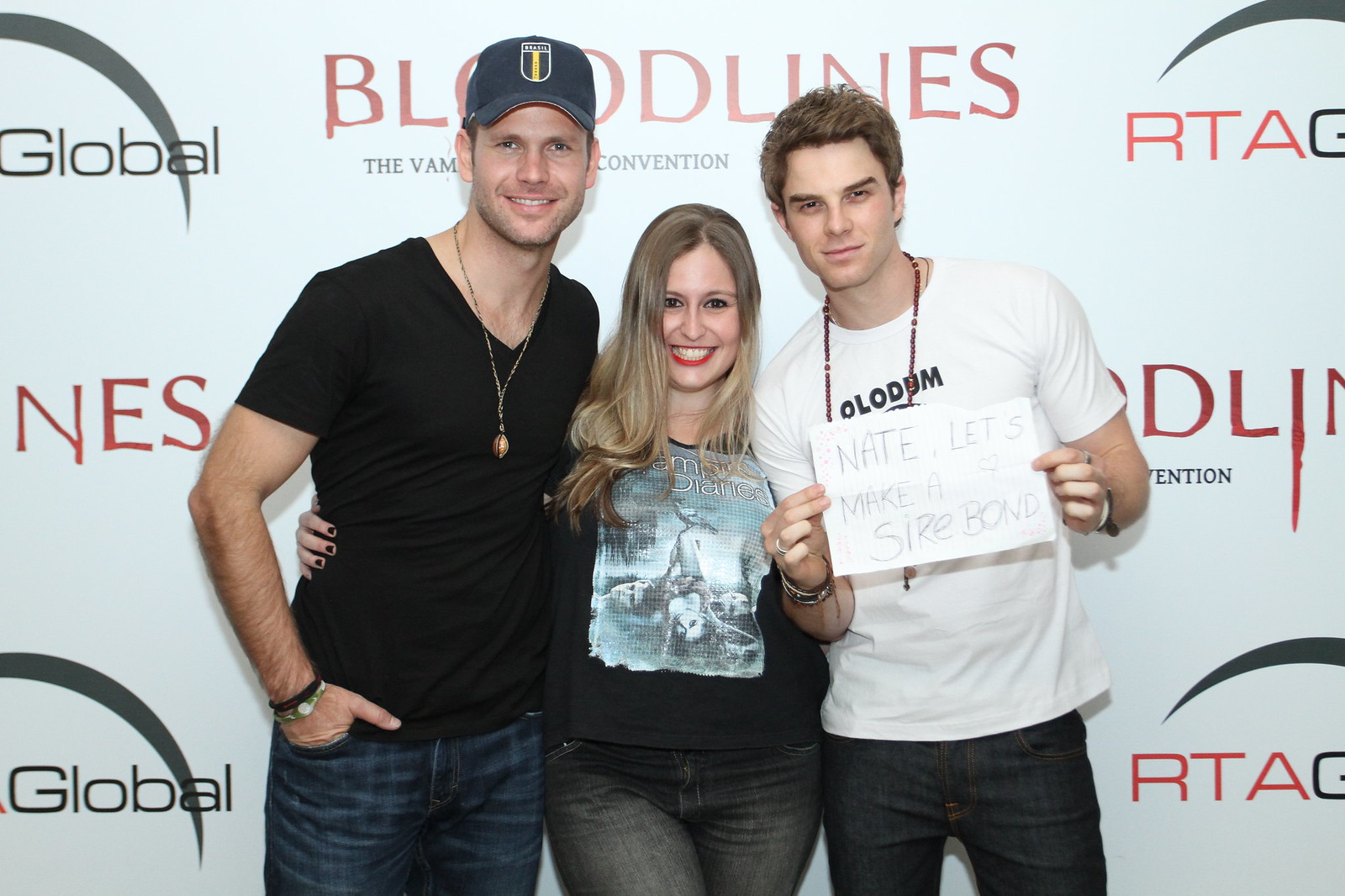In this vibrant photo taken at a Bloodlines, The Vampire Diaries event, fans are seen enthusiastically greeting actors amidst a dynamic backdrop. On the far left, a man wearing a black t-shirt and a baseball cap stands beside a woman proudly donning a Vampire Diaries t-shirt and blue jeans. Together, they are joined by another man on the right who holds a striking sign that reads, "Nate, let's make a sire bond." The trio stands in front of a white background adorned with black and red lettering, showcasing the Bloodlines sponsorship logos and advertisements for The Vampire Convention. Prominent in the scene is actor Paul Wesley, who is mingling with the fans, further enriching this special moment at the red carpet-like meet and greet event.